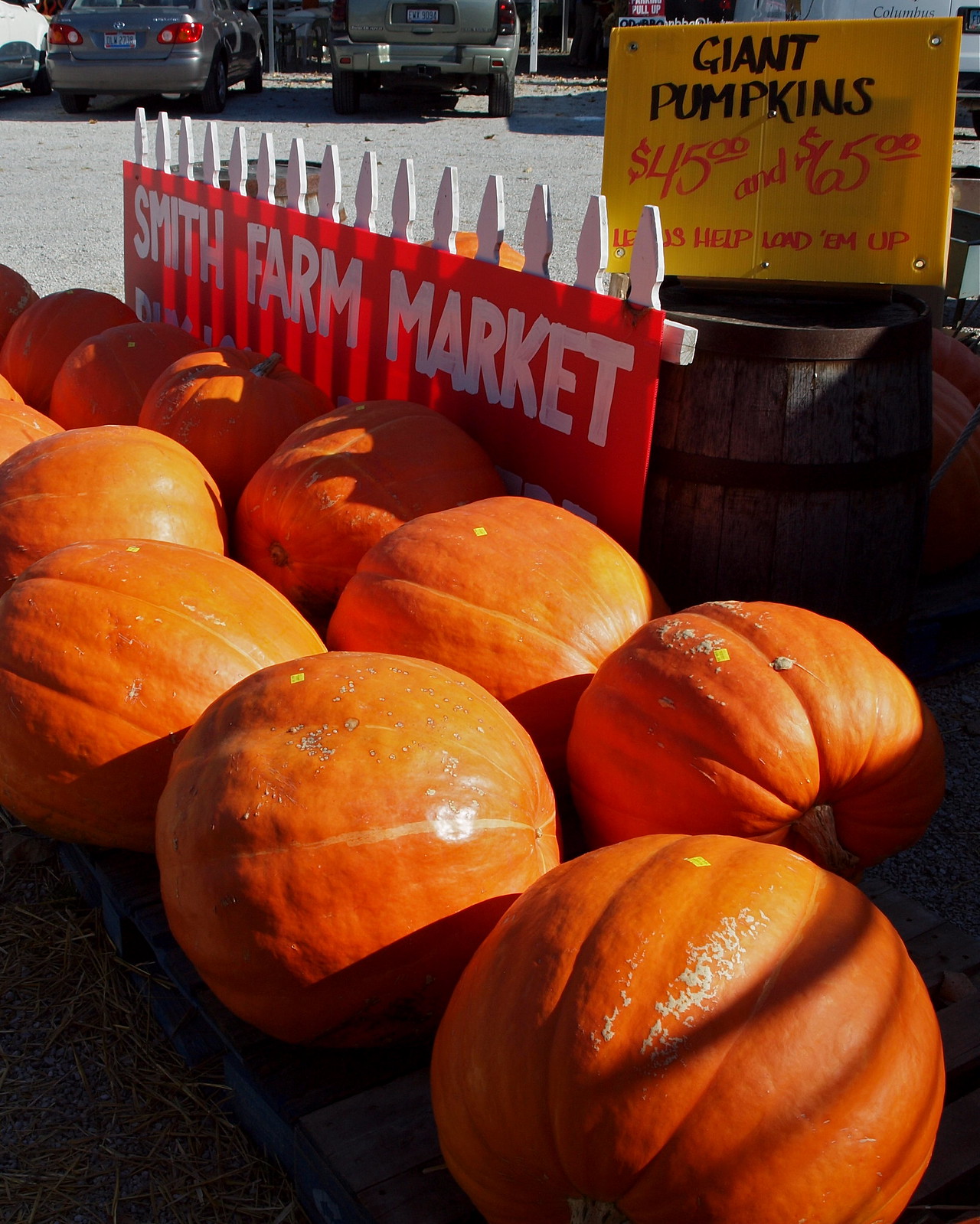The photograph captures the vibrant entrance of Smith Farm Market, characterized by a prominent white picket fence adorned with a bold red sign that reads "Smith Farm Market" in white lettering. In the foreground, two rows of impressively large orange pumpkins are on display—four in the front row and about six in the back. Positioned behind these pumpkins is a rustic wooden barrel, reinforced with metal bands. Atop the barrel, a yellow sign highlights the sale of "Giant Pumpkins" in striking black and red text, listing prices of $45.00 and $65.00, followed by additional, partially obscured, red text that hints at assistance for loading. The scene is set beside a parking lot, with noticeable vehicles, including a gray car and a darker gray car, providing a practical backdrop to the lively market atmosphere.